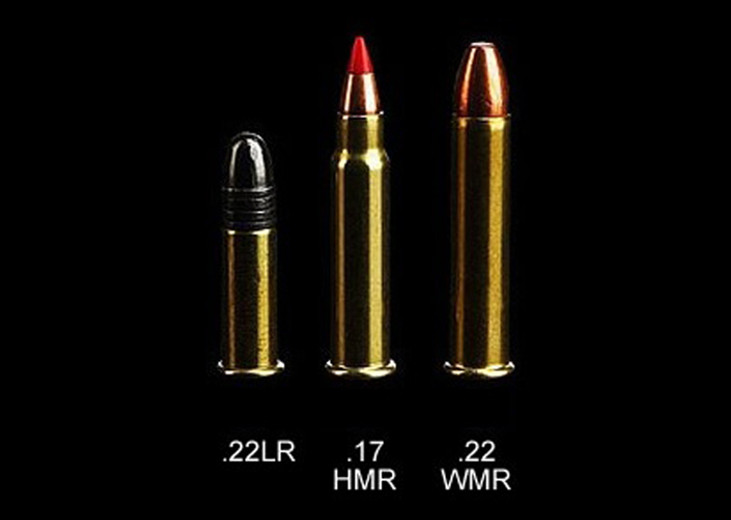The image features three different calibers of bullets against a solid black background, each centered vertically with white text beneath them indicating their respective calibers. The first bullet on the left is labeled ".22 LR" and is the shortest, featuring a gold casing with a rounded black tip that has lines down it. The middle bullet, labeled ".17 HMR", is the tallest, with a longer gold casing and a pointed tip that's bright red at the top and copper-colored below the red tip. The third bullet on the right is labeled ".22 WMR" and has a wider base. It's slightly shorter than the middle bullet and features a gold casing with a flattened, rounded darker gold tip.